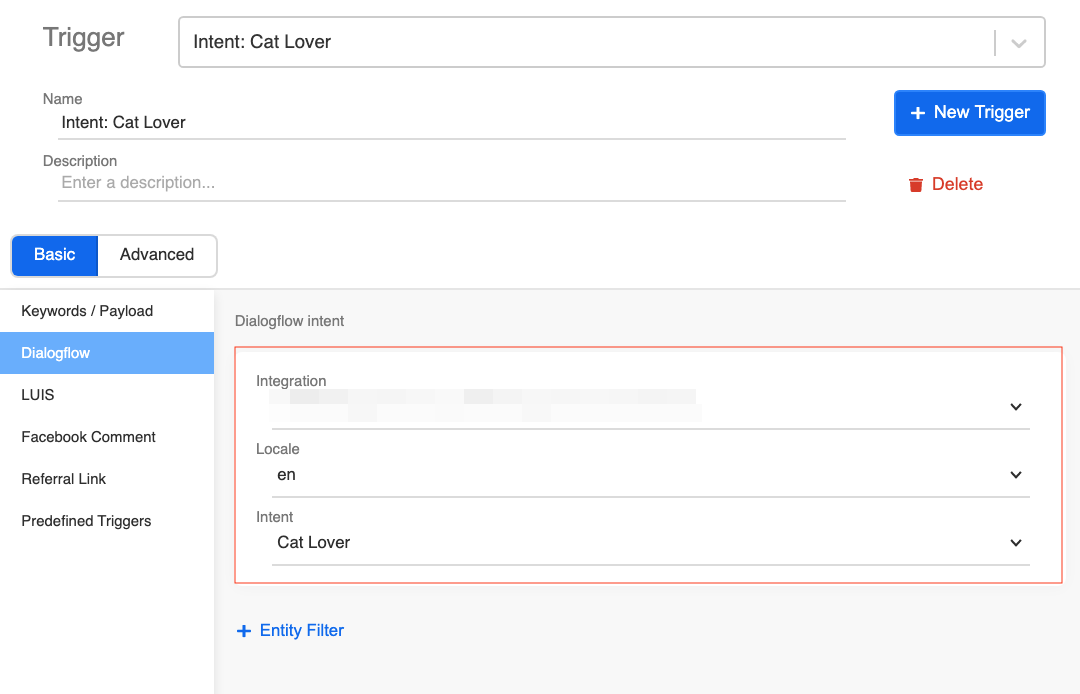The image depicts a user interface for configuring triggers in a conversational AI platform. At the top of the screen, there is a line labeled “Trigger” with an adjacent drop-down list where "intent: cat lover" is the selected option. Following this, another line labeled “Name” displays "intent: cat lover." A button labeled "+ New Trigger" is also visible.

Below this, there is a description field that is currently empty, alongside a delete icon represented by a small garbage can icon and the text "Delete."

A toggle selection button is present, offering options "Basic" and "Advanced," with "Basic" being selected. 

The content area of the page is divided into two main sections. The left column contains a list of keyword payload options, with "dialogflow" being the selected choice. Other options listed include LUIS, Facebook comment, referral link, and predefined triggers.

On the right side, under a section heading labeled "Dialogflow Intent," there is a box outlined in red containing several drop-down lists. The first drop-down is labeled "Integration," but no option is selected. The second drop-down, labeled "Locale," has "EN" selected. The third drop-down, labeled "Intent," has "Cat Lover" selected. At the bottom of this section, there is a button labeled "+ Entity Filler."

The interface appears to be a structured and organized environment for managing various triggers, intents, and integrations for a dialog or chatbot system.